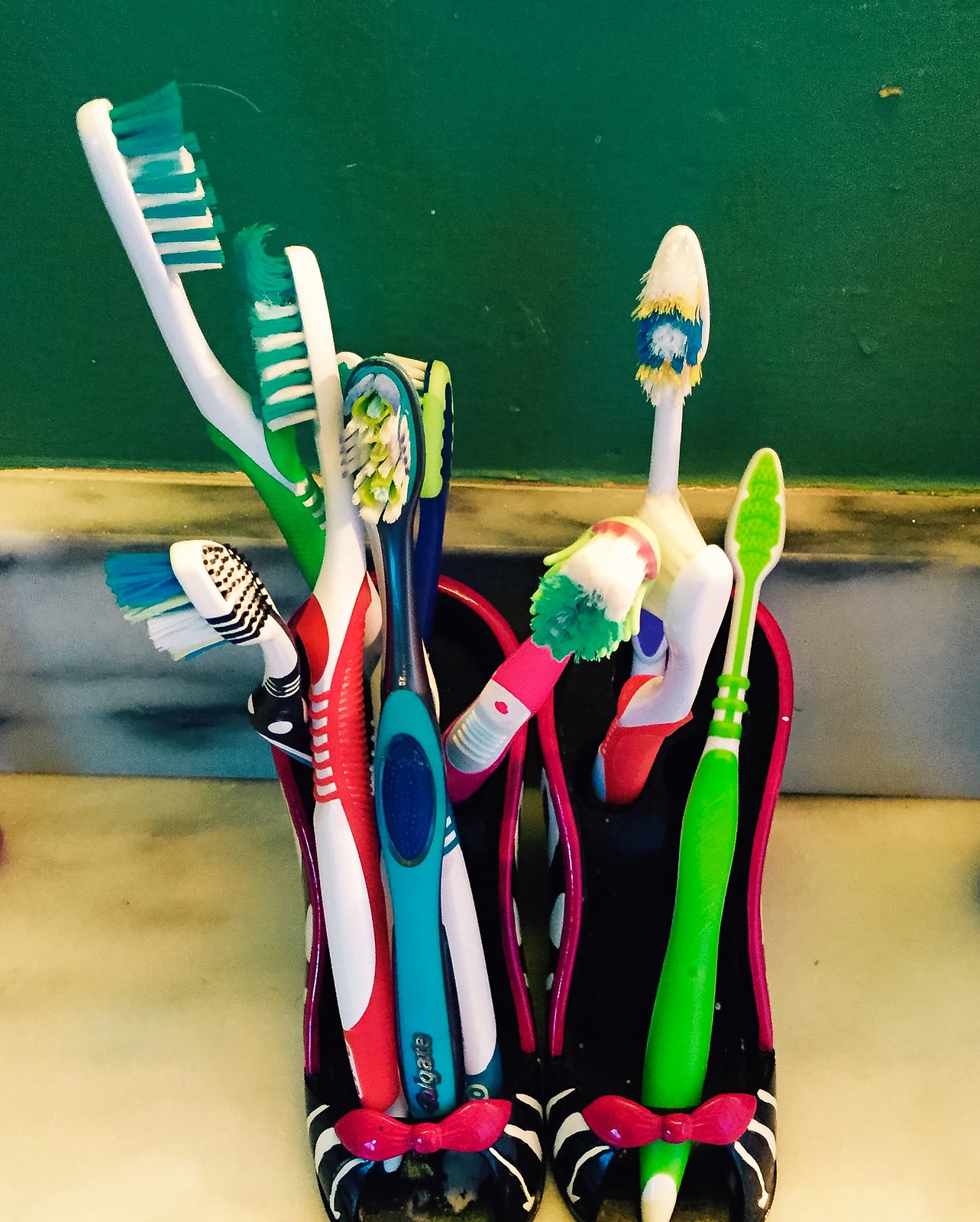This color photograph features a quirky and detailed scene of two black ceramic high-heeled shoes being used creatively as toothbrush holders. Each shoe is designed with pink bows near the open toes, white stripes across the toe area, and a pink outline around the opening. The shoes, resembling women's high-heeled pumps, are filled with a total of nine toothbrushes, showcasing a variety of colors and styles. The left shoe contains six toothbrushes in multicolored shades including pink, blue, green, and black, with bristles jutting out in different directions. The right shoe holds three toothbrushes: one green, one red, white, and blue that appears crooked, and a third one with blue, yellow, and white bristles. The background is a mix of deep green and grey, with a wooden texture at the top that features black markings. The shoes rest on a beige surface, completing this whimsical and visually engaging setup.